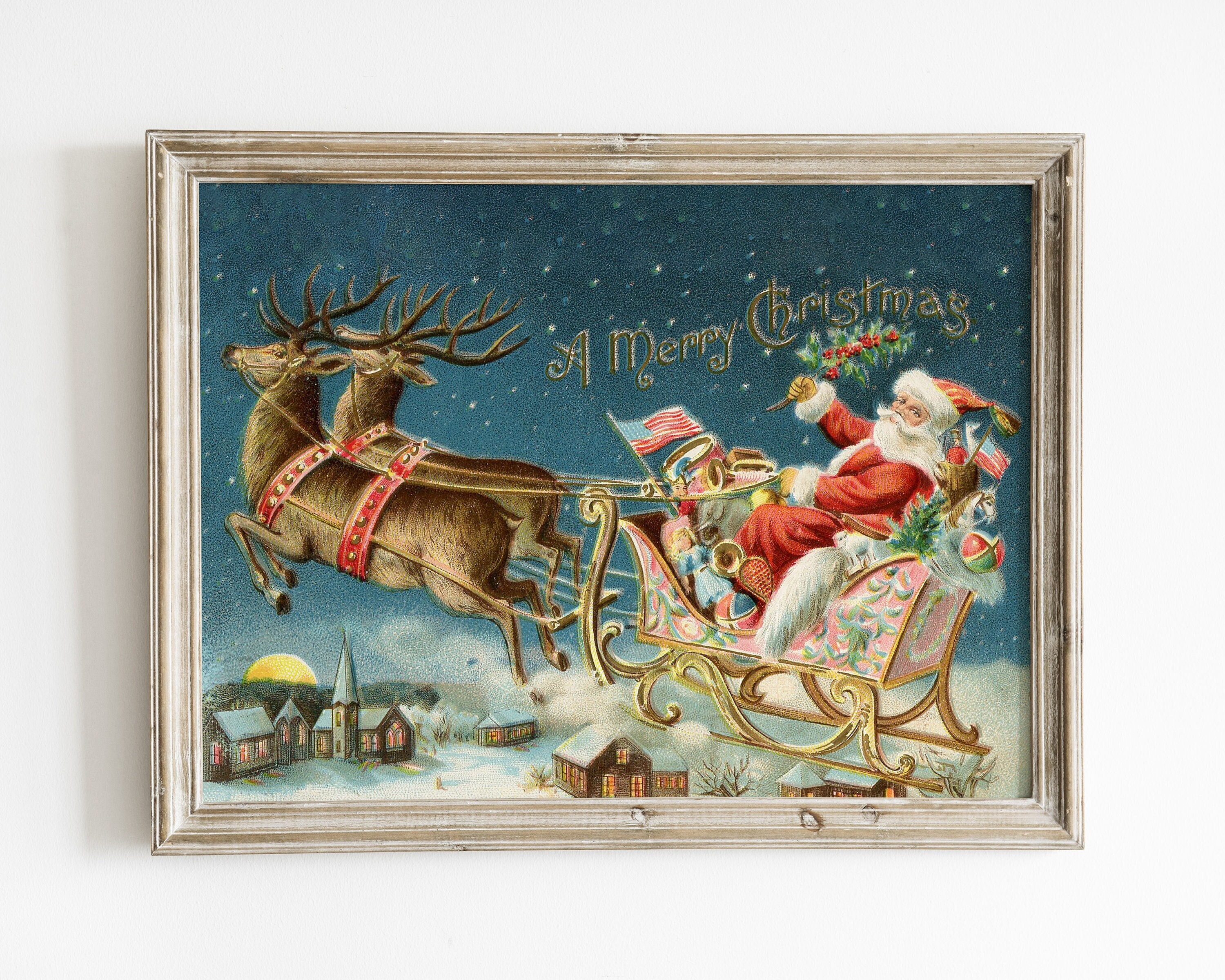This detailed image in a picture frame hangs on a white wall. The frame itself is a lightly painted wood, possibly light silver or goldish in hue. The artistic drawing within captures a festive night sky filled with either stars or snowflakes. Centered in the image is a pinkish sleigh trimmed in gold, piloted by Santa Claus in his traditional red attire with white cuffs. In his left hand, Santa holds the reins of two reindeer adorned with red harnesses and gold bells, guiding them through the sky. His right hand clutches holly, and an American flag is prominently displayed on the sleigh. Scattered around Santa are various toys, emphasizing the Christmas spirit. Above Santa in elegant golden cursive, the words "A Merry Christmas" are inscribed. Beneath this sky scene lies a cozy, snow-covered village, complete with houses and a church, their lights glowing softly. The moon rests on the horizon just behind the quaint town, completing the serene wintry landscape.